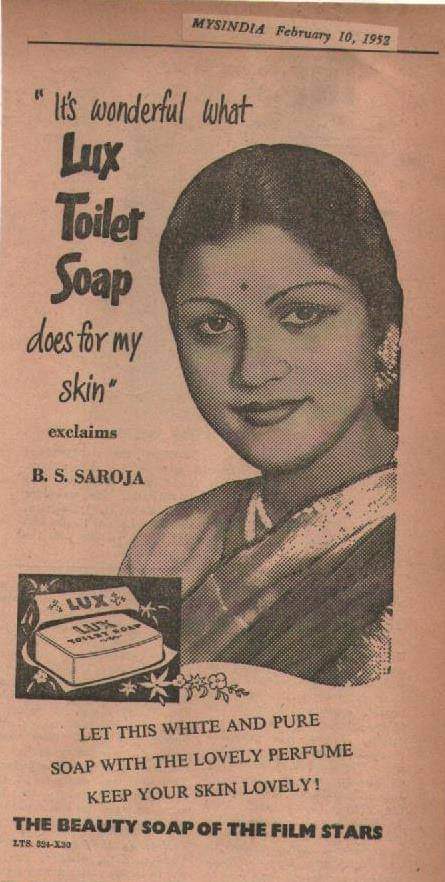This detailed advertisement from February 10th, 1952, showcases Lux Toilet Soap, endorsed by Miss India, B. S. Siraja. The vintage ad, which has aged to a brownish hue and contains some watermarks, features a black-and-white photograph of an Indian woman with her hair pulled back and a traditional dot on her forehead. She wears a sari that appears shiny, almost gold-like. The ad prominently displays the tagline, "It's wonderful what Lux Toilet Soap does for my skin," highlighting the soap's pure and white quality with a lovely perfume that promises to keep your skin radiant. The illustration of the Lux soap bar further emphasizes the product, aiming to evoke a sense of luxury and effectiveness. The overall appearance and text underscore the soap's timeless appeal and superior cleansing properties.